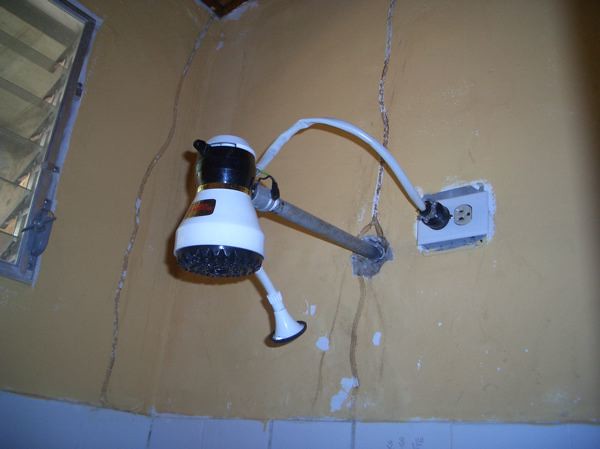The image depicts a cluttered, somewhat dilapidated bathroom. At the center is a horizontal, gray metal pole protruding from the cream-colored, cracking plaster wall, which supports a peculiar device reminiscent of a shower head. This device features a black and white body with an upside-down, flowerpot shape, and a black and red label. It is plugged into a nearby electrical socket, posing an unusual and potentially hazardous setup. The wall bears long, noticeable cracks and appears partially painted with blue splotches along the bottom and around the power socket, indicating wear and neglect.

On the left side of the image is an old-style glass pane window with partially open gray shutters, contributing to the room's run-down appearance. Below the metallic pole and device, white bathroom tiles can be seen, dividing the upper cream wall from the lower tiled section. Additionally, there's a prominent vent with aluminum louvers that looks like it can facilitate airflow, though the general condition of the room suggests infrequent maintenance. The overall ambiance is one of dereliction, contrasting starkly with the somewhat new-looking shower head-like device plugged into the wall.